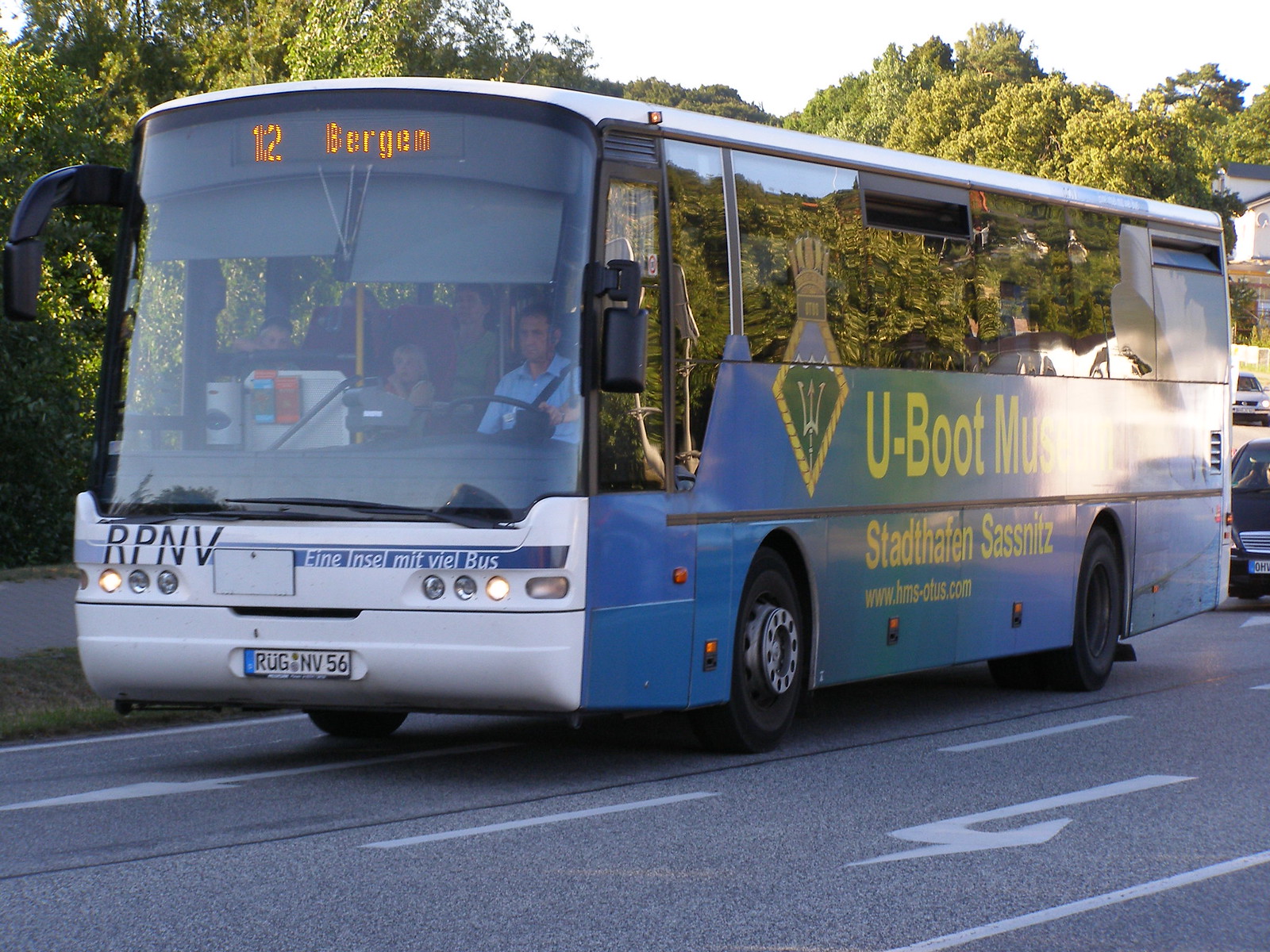This photograph captures a blue and white bus traveling on a sunny day on a highway, flanked by green trees illuminated by the sunlight. The road is smooth and has white lane markers and arrows, signaling an upcoming left turn. The bus is prominently featured, facing towards the camera, with its lights turned on and a license plate reading "R-U-G-N-V-56." The front LED display of the bus shows the route number "12" and the destination "Bergen." The bus carries additional text in what appears to be German, including phrases like “U-Boot Museum,” “Stadthafen, Sassnitz,” and “Ein Insel mit Viele Bus.”

The driver's side of the bus, with the steering wheel on the left, shows a male driver in a blue uniform, buckled in. The reflective windows reveal a glimpse of passengers, including a blonde girl behind the driver and possibly an adult next to her. The side of the bus has a diamond-shaped logo featuring a golden trident on a green and white field. The entire scene is bathed in natural sunlight, suggesting a clear, bright day. This composition emphasizes the serene, orderly setting, highlighting the bus in its route through a scenic and well-maintained roadway.